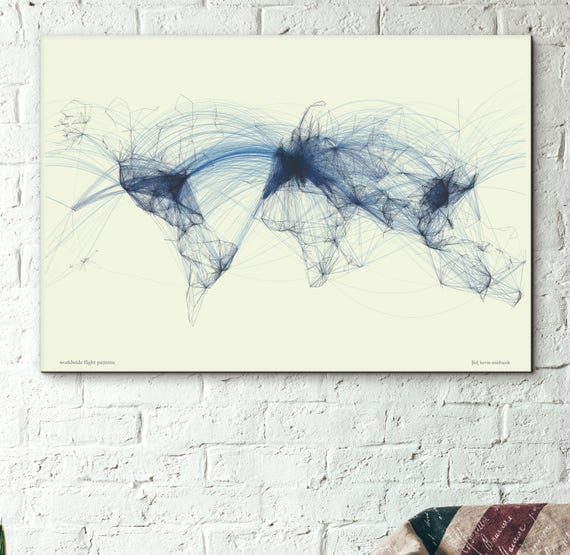The image showcases an abstract illustration of the world map on a white-painted brick wall, blending modern and distressed elements. The map utilizes black and dark blue lines that appear to represent flight patterns or logs, with notable emphasis on North America, Europe, and Eastern Asia. The intricate line art features various pen-like strokes radiating between the continents, creating an interconnected, atmospheric effect. In the bottom right corner, there is part of a couch adorned with tan, dark red, and dark green stripes, along with cursive writing, adding a touch of color and texture to the scene. Additionally, there are watermarks visible on the bottom left and right-hand sides of the print.